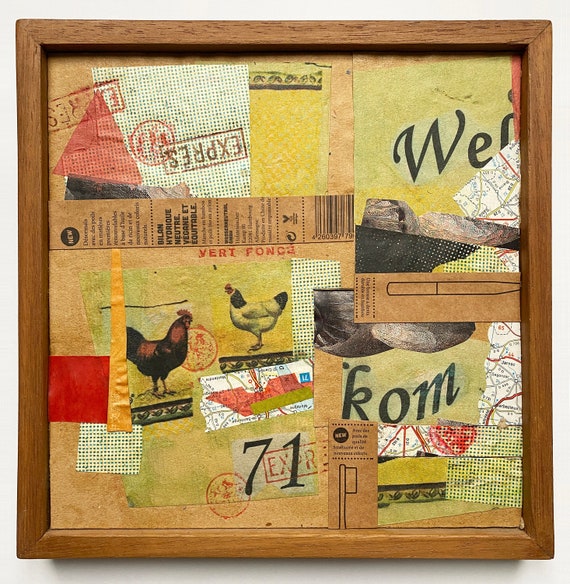The image features a framed art piece, elegantly mounted within a medium-light brown wooden frame, slightly polished with hints of black grain, and shaped square. The artwork showcases an intricate collage constructed from various paper cutouts, resembling pieces from letters, postcards, and newspapers. Dominating the center is a square cutout depicting two roosters. The collage incorporates multiple elements, including a beige and yellowish color palette with touches of white, a textured feel suggestive of fabric swatches, and an assortment of stamps and printed letters. Notably, there is an upside-down stamp bearing the word "EXPRES," the letters "W-E-L" in the upper right, the cutout square featuring the number "71" towards the bottom, and the phrase "VERT FONCE." Additionally, "K-O-M" appears prominently. A piece of a map and various ink stampings, particularly one in red, further enhance the eclectic and unique design of this kitchen-friendly artwork.